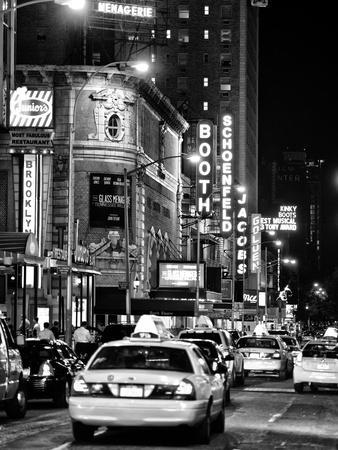A black-and-white photograph captures a bustling New York City street scene, likely from the 1930s or 1940s. The image, taken at night as evidenced by the glowing lights and dark sky, showcases a crowded road, full of vintage taxis identifiable by their rooftop signs. The sidewalks teem with people. Prominent, illuminated vertical and horizontal signs on the buildings advertise various businesses and Broadway shows. Notable signs include "Brooklyn," "Booth," "Schoenfeld," "Jacobs," "Glass Menagerie," and more. In the distance, the silhouettes of towering high-rise buildings frame the scene. Bright lights and numerous billboards filled with advertisements contribute to the lively atmosphere of this historic urban setting.